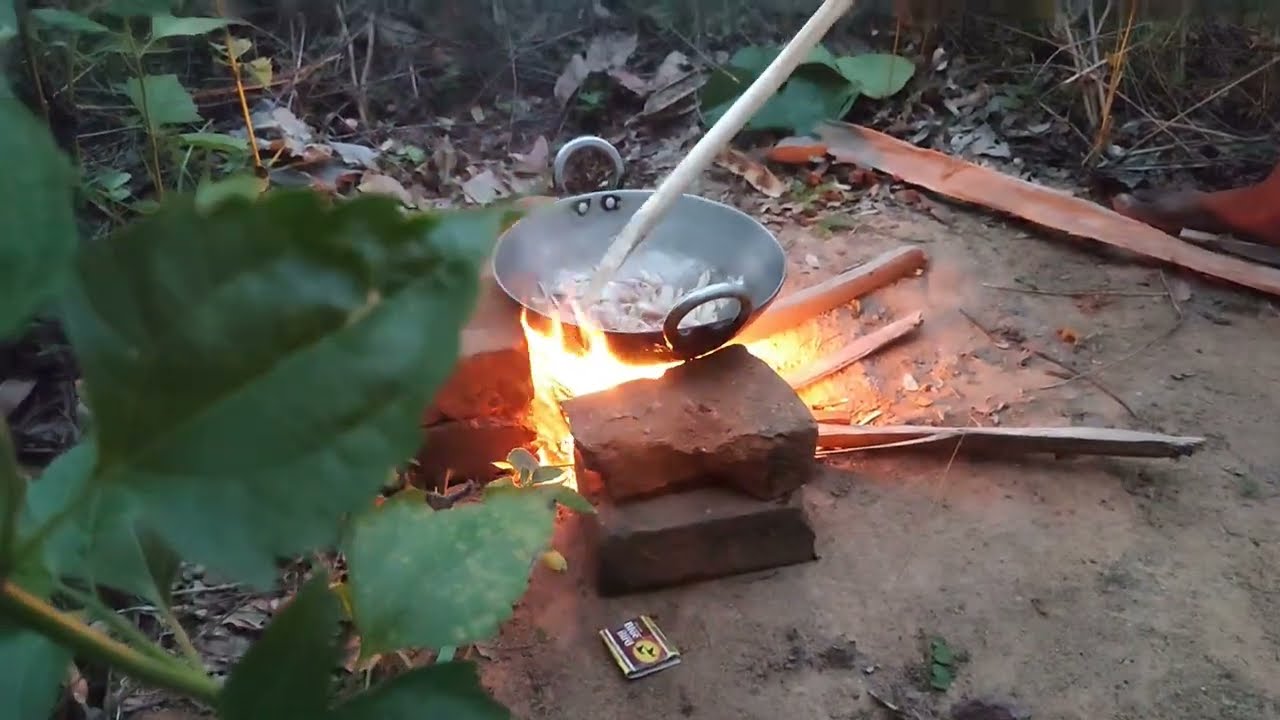In this outdoor photograph, a rustic campfire cooking setup is showcased in a natural environment. The foreground features wet, muddy soil bordered by green foliage, dried leaves, grasses, and tree bark. At the image's center, a makeshift fire pit, crafted from stacked bricks, contains a small, dug-out pit filled with kindling and twigs, engulfed in a glowing, orange flame. Positioned atop the brick structure is a large two-handled wok, made of shiny metal, with visible food being stirred by a long handle inserted within. Scattered around the scene are matches, more twigs, and branches, providing additional context and emphasizing the rough, yet purposeful, nature of this outdoor cooking endeavor.